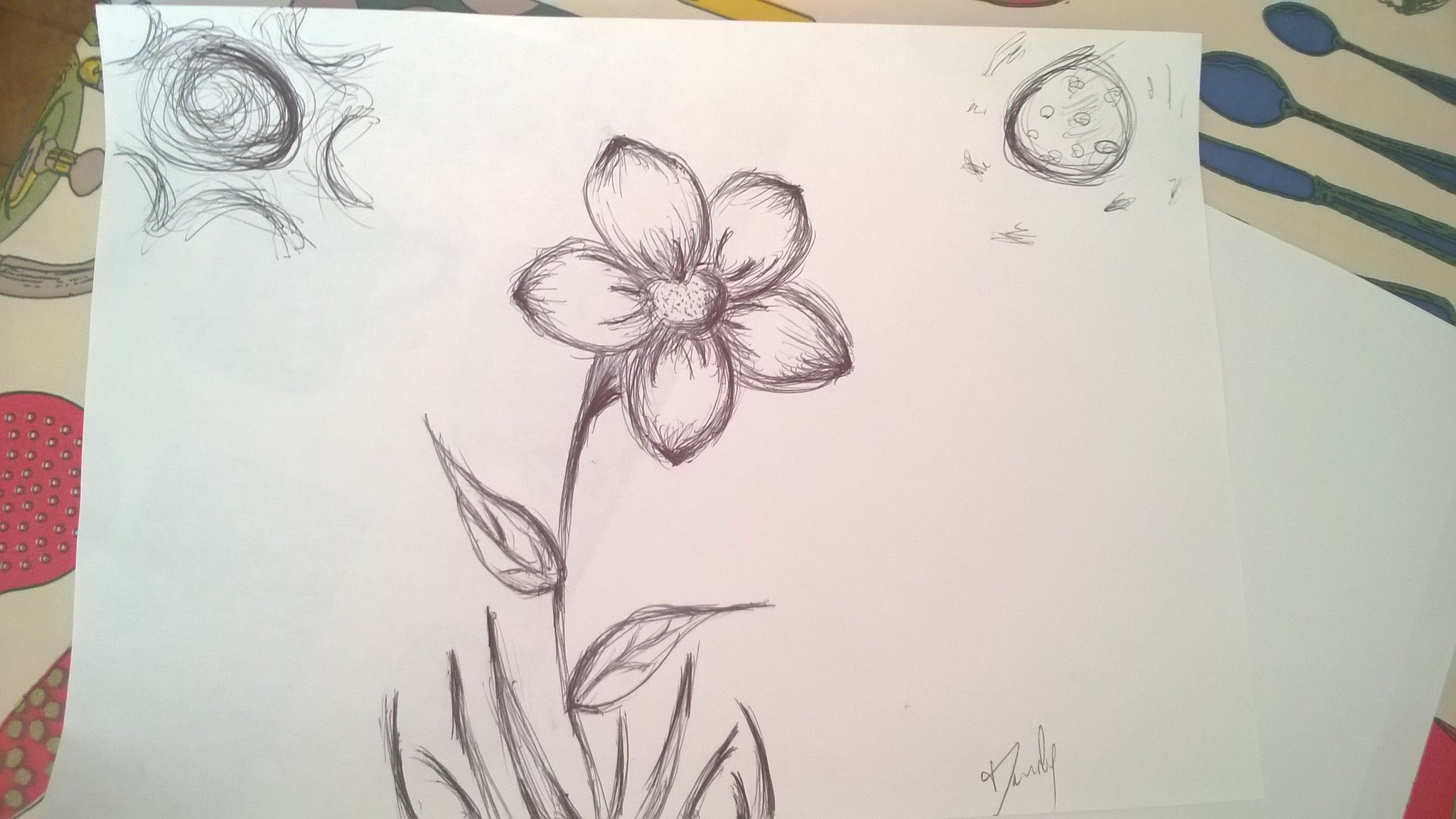In this color photo, a piece of white printer paper rests atop a table adorned with a decorative tablecloth featuring blue cutlery and fruit motifs. The paper showcases a series of intricate pen and ink drawings, all in black and white. Positioned in the upper left corner is a finely detailed sun, its rays meticulously rendered. Directly opposing it in the upper right corner is an image of a moon, distinguished by crater-like textures that add depth to its portrayal. Dominating the center of the sheet is a striking illustration of a five-petaled flower, complete with a clearly defined pistil and stamen. The flower's stem is flanked by two asymmetrical leaves, one higher than the other, and beneath these are blades of grass that provide a grounding element. Completing this artistic composition is the artist's cursive signature, located at the bottom right of the page, which appears to read "Darby."